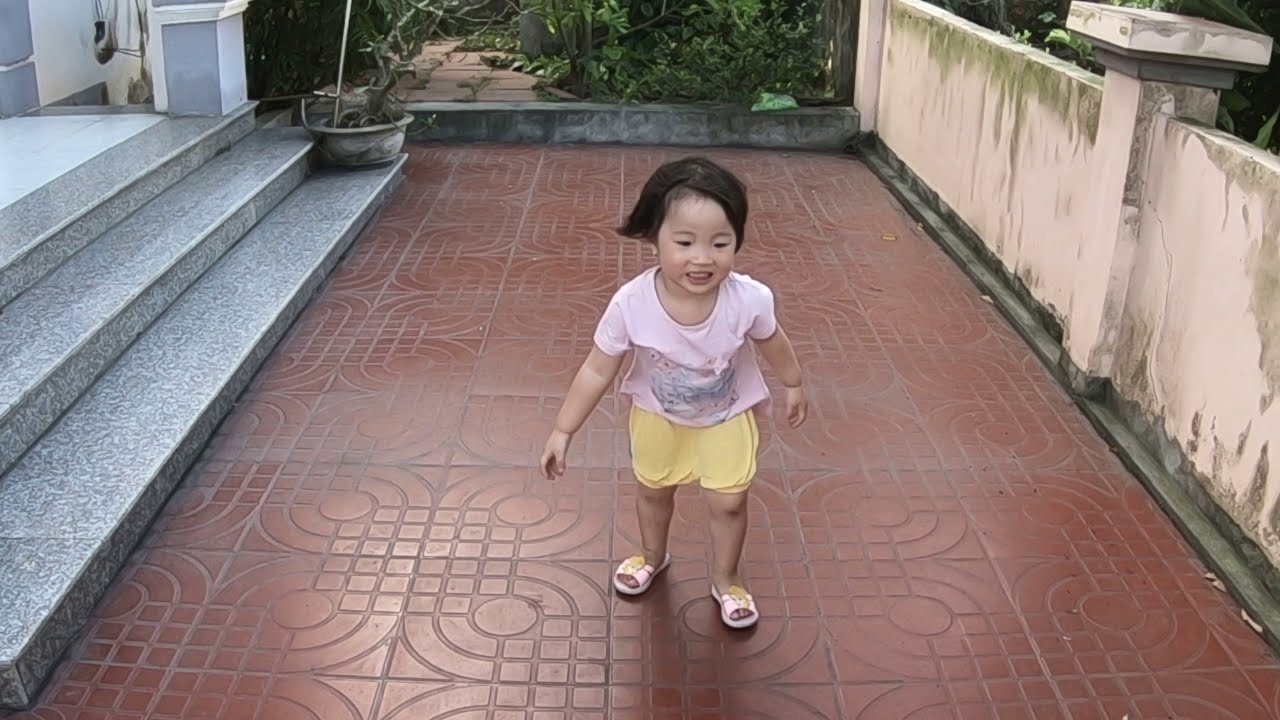The image captures a young Asian girl, approximately 3 or 4 years old, standing at the forefront of a decorative patio. She is dressed in a light pink shirt adorned with a subtle design, yellow shorts, and light pink sandals. Her black hair contrasts with her lighter skin complexion, and she wears a cheerful smile while looking downwards. The ground beneath her features a maroonish tile with unique diamond and circular inscriptions. On her left side are speckled gray and white granite steps, possibly leading into a house, while on her right, a slightly dilapidated concrete wall stained with green mildew runs parallel to her. Above her and in the background, there are plants and a step potentially leading to another section of the outdoor area, bathed in ample natural daylight that indicates the photo was taken during the day.